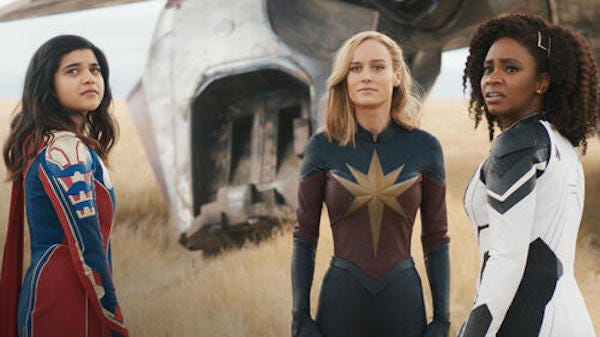This image is a detailed still shot from the movie "Marvels," featuring three women dressed as superheroes standing in a field of tan, dead grass. On the left, a young woman with long dark brown hair is seen turning her body to the right while looking back over her shoulder, and she's dressed in a predominantly red and blue costume with white accents and a red cape. In the middle, a blonde woman with shoulder-length hair faces forward, wearing a dark blue and dark red costume adorned with a spiky gold star on her chest. On the right, a woman of African descent with black curly hair and dark skin is shown in a white costume with black details, her head turned to gaze over the viewer's left shoulder. The background features a crashed metallic structure, resembling a silver or gray spaceship, set against the yellow hues of the field.